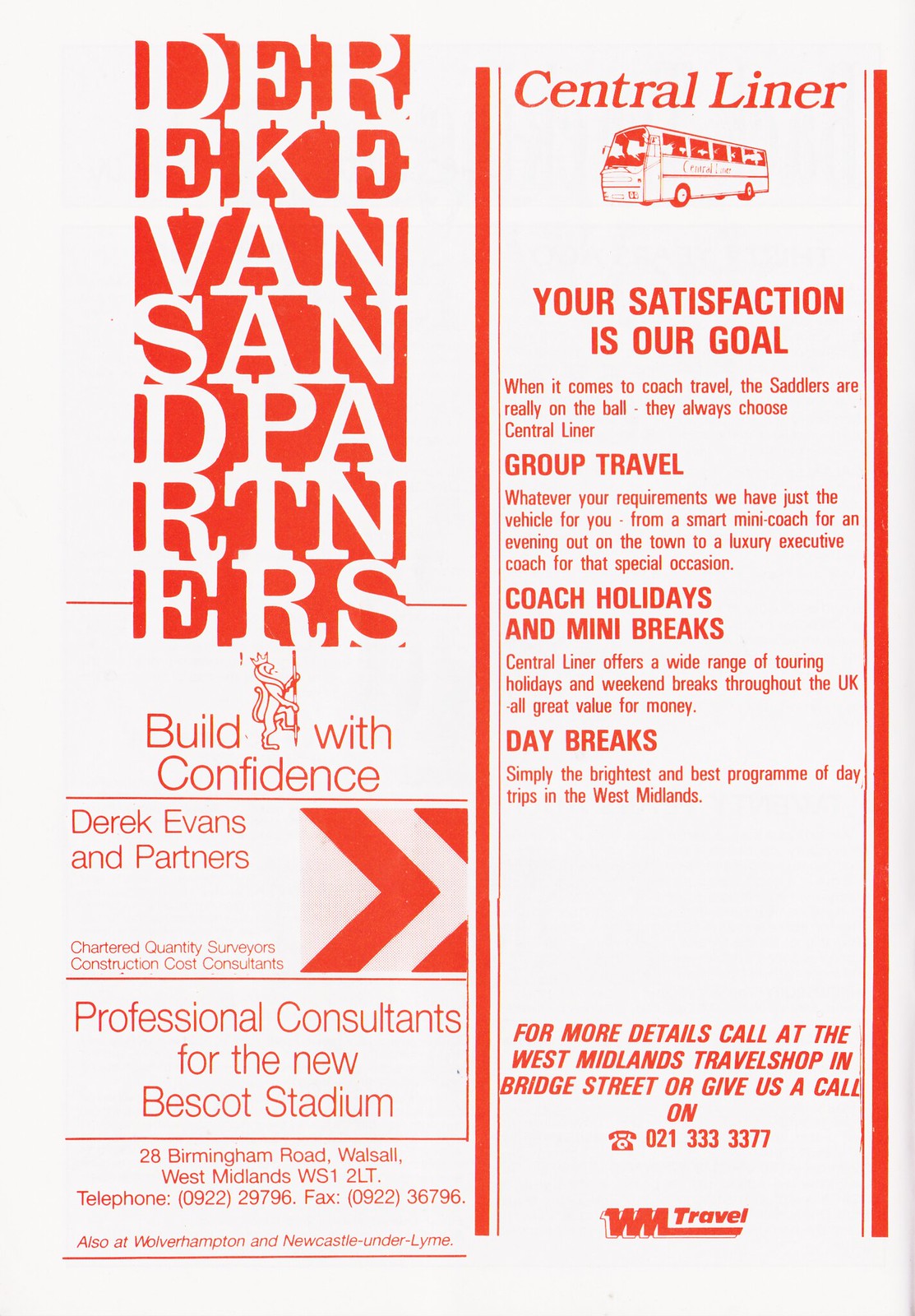The advertisement is aesthetically minimalistic with a light blue background and prominently uses red text to convey its message. The page is divided into two vertical columns.

On the left column, a large red rectangle features white stenciled letters stacked vertically. From top to bottom, these letters read: DER, EKE, VAN, SAN, DPA, RTN, ERS. Below this rectangular panel, the text reads: "Build with Confidence." This is followed by "Derek Evans and Partners, Chartered Quarterly Surveyors, Construction Cost Consultants, Professional Consultants for the New Bescott Stadium." The address and contact details are listed as: "26 Birmingham Road, Walsall, West Midlands, WS12LT. Telephone 0922-29796, Fax 0922-36796."

The right column features the heading "Central Liner," along with a sketched graphic of a bus or trolley. Beneath this, it states: "Your satisfaction is our goal. When it comes to coach travel, the Sadlers are really on the ball; they always choose Central Liner." It elaborates on their services: "Group travel, whatever your requirements, we have just the vehicle for you—from a smart mini coach for an evening out on the town to a luxury executive coach for that special occasion. Coach holidays and mini breaks, Central Liner offers a wide range of touring holidays and weekend breaks throughout the UK, all great value for money." Furthermore, it mentions "Day breaks: These are the brightest and best programs of day trips in the West Midlands." For additional details, it suggests contacting the West Midlands Travel Shop in Bridge Street or calling 021-333-3377. The logo of WM Travel is displayed at the bottom of the page.